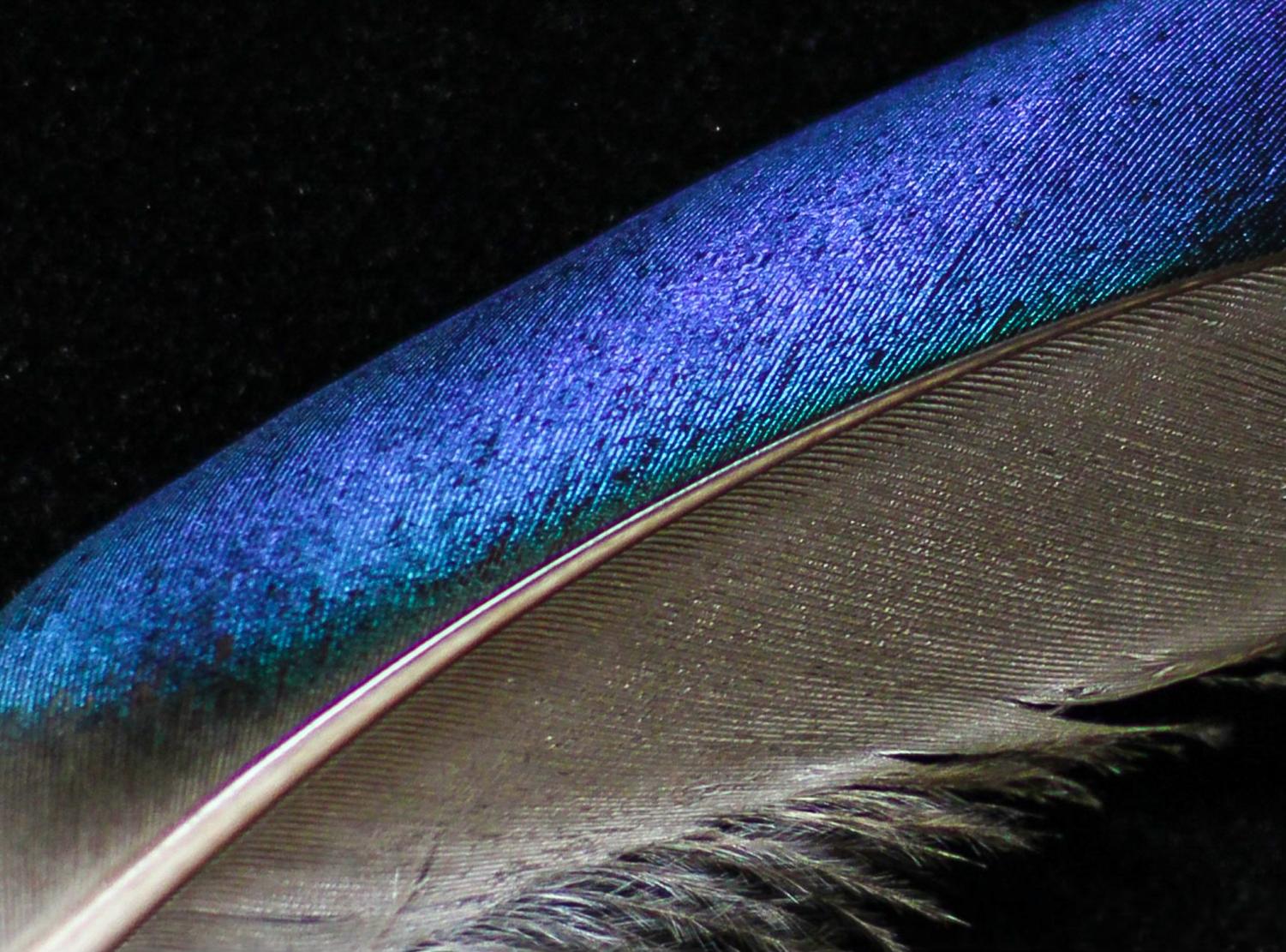In this detailed close-up photo, a single feather dominates the composition, set against a stark black background. The feather extends diagonally from the lower left to the upper right corner of the frame. The feather is split into two distinct sections: the lower segment is an iridescent gray with loose, feathery fibers, and the upper portion is a vibrant iridescent bluish-purple. The feather's intricate structure is visible, with individual lines or barbs clearly distinguishable. At the lower end, these barbs spread out more loosely, creating a slightly frayed appearance. As they ascend, they align more diagonally, particularly in the blue section, adding to the feather’s delicate, yet complex, beauty.